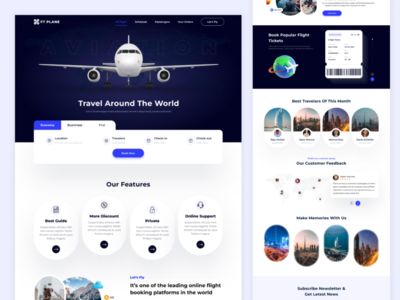This composite image showcases two website mockups side by side. The first mockup, framed by a pale purple-gray border on all sides except the bottom, features a night sky scene with a flying airplane and the text "Travel Around the World." Beneath this, a gradient background transitions from blue to purple to bright white, adorned with an unreadable blurred section containing a small banner and a pushable button or tab. Below this, four oval elements, each containing an icon and bold, yet blurred and unreadable text, are arranged in a row.

On the right side, the second mockup resembles a smartphone interface. It mirrors the night sky background and includes an image of a globe with a plane circling it. This mockup also features a tab or barcode section, flanked by additional images and text at the top and bottom, all of which are blurred and unreadable. The overall design hints at a travel-themed digital interface, although the specific details remain unclear due to the blurred text.